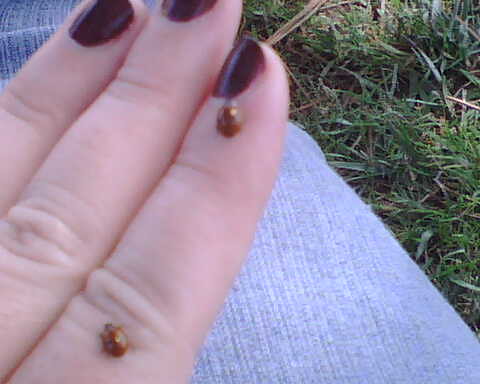In a close-up, slightly grainy image, three fingers of a woman's right hand are prominently featured. She has thick, light-skinned fingers adorned with brown-maroon nail polish, and only her index, middle, and ring fingers are visible. On her index finger, at the tip by her fingernail, perches a golden ladybug. Another golden ladybug is positioned on her index finger's knuckle. The background reveals she's outdoors, wearing blue denim jeans and sitting on grass that is primarily green with some brown specks, likely twigs. The photograph is so zoomed in that the tip of her middle finger is cut off by the frame. The image orientation suggests her hand is angled diagonally.